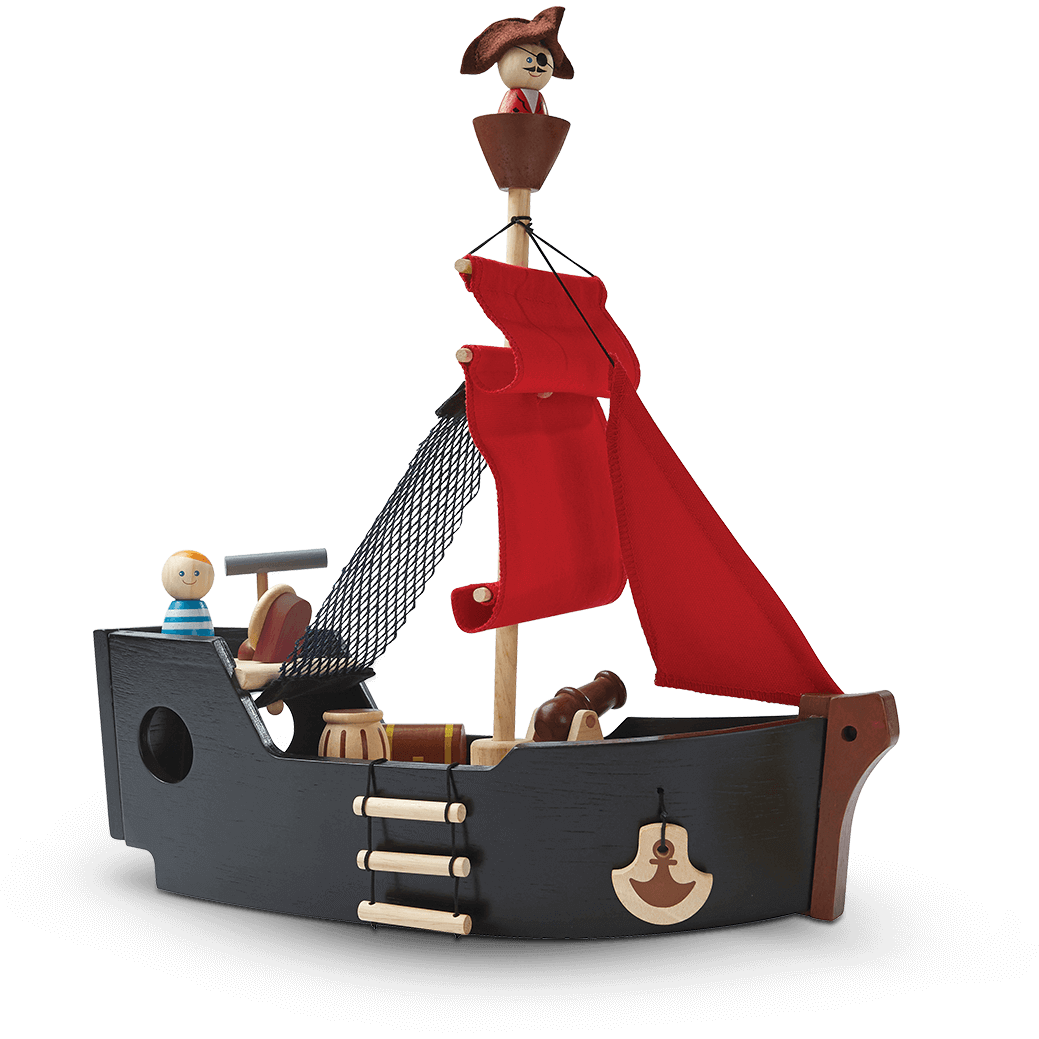The image showcases a detailed wooden toy pirate ship centered against a plain white background. The ship itself features a blue body with brown trim, and it is equipped with a single mast that supports two red sails and a crow's nest at the top. A pirate figure resides in the crow's nest, identifiable by a black eye patch, a mustache, and a red-and-white top with a pirate hat. Below on the deck, another small wooden figure with orange hair, a blue-and-white outfit, and a smiling face stands to the left, likely representing a first mate. The ship is adorned with various pirate-themed elements, such as a wooden ladder, a cannon on the right side, a barrel on the left side, a treasure chest, and a small anchor hanging from the side. The intricate details and array of accessories contribute to the ship's charming pirate aesthetic.